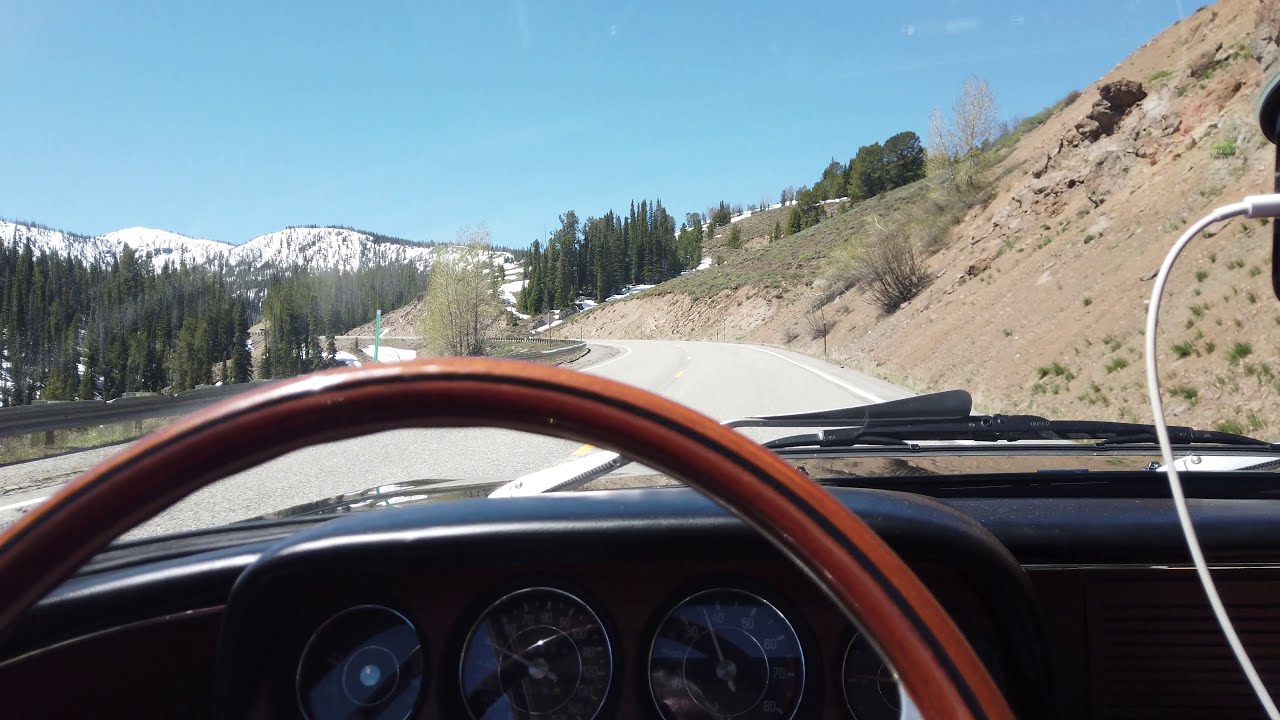A vintage car, seemingly from the 70s or 80s, is captured from the driver's seat as it navigates a winding, hilly road. The interior features a leather red steering wheel with a black stripe running through its center and a non-digital dashboard with visible speedometer and odometer. The black dashboard also shows a USB charger and an iPhone cable plugged into an unseen device. Outside the windshield, the paved road curls gracefully towards snow-capped mountains under a clear, crisp blue sky with hardly any clouds. On the right side of the road, lightly grassed, sandy hills suggest a potential for landslides, shifting into a landscape of lush green trees and patches of snow as the car heads further along. The highway is split, with the opposite direction at a slightly lower altitude. Evergreen trees dot the scene, complementing the serene, sunlit day that feels like the tail end of winter or early spring, where bits of melting snow are scattered between the trees.